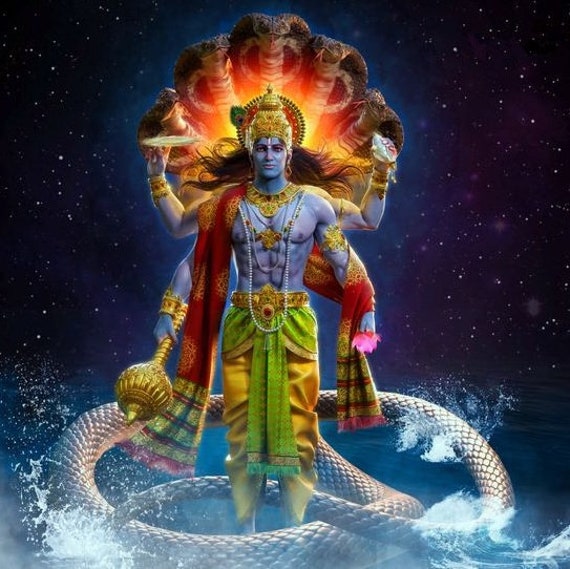In this stylized photograph, a mystical, blue-skinned deity stands against a starry, black, and purple background dotted with white stars. This powerful figure is shirtless, revealing a muscular torso of pale blue to lavender hues. His long brown hair flows beneath an ornate golden headpiece, and additional golden adornments include a detailed band around his waist, which is also decorated with a red gem. He wears yellow pants combined with green fabric near the waist, complemented by a green loincloth. A striking red scarf drapes over his right shoulder, loops around his left arm, and cascades down his back.

The deity possesses four arms, each holding symbolic items: a large, golden scepter with a bulbous top in his right front hand, a pink flower in his left front hand, a blue gem or stone in his left rear hand, and a spiral galaxy balanced on his right rear hand. His right forearm is further adorned with a gold band.

Behind him, a striking halo of five snakes emerges, the central and largest being a dark cobra, flanked by two cobras on each side. Below, the body and tail of one of these serpents twist ominously around his feet, surging from a bottom row accented by splashes of white water.

The celestial setting, with its rich palette of vibrant colors, underscores the deity's mystical and powerful presence.